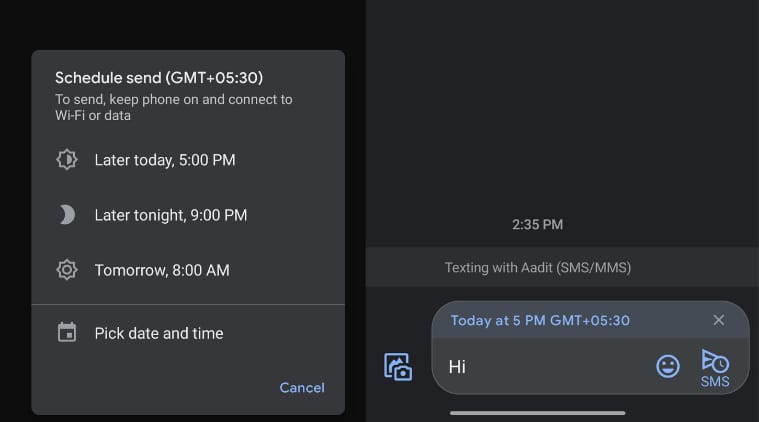The image features a user interface on a black background, divided into two main sections in a horizontal layout. 

**Left Section:**
- Titled "Schedule Send" with the time noted as "GMT+05:30."
- Instructions inform the user to keep their phone on and connected to Wi-Fi or data to send the message.
- Options are listed for scheduling the message:
  - Later today at 5 p.m.
  - Later tonight at 9 p.m.
  - Tomorrow at 8 a.m.
- A thin separator line followed by the option to "Pick day and time."
- A "Cancel" button appears in blue in the top right corner of this section.

**Right Section:**
- Shows the current time as "2:35 p.m."
- Indicates that it is "Texting with Adit" (noted as SMS/MMS).
- States a scheduled send time for "Today at 5 p.m. GMT+05:30" in blue text.
- Below this, there is a text field containing the message "Hi."
- Features icons for emojis, a clock, and an SMS button (depicted as an enter button or right arrow) in blue.
- To the left outside the text field, there is a camera icon also in blue.

This division of content and careful detailing suggest it's from a messaging app interface, highlighting how to schedule messages and the status of the message scheduling process.